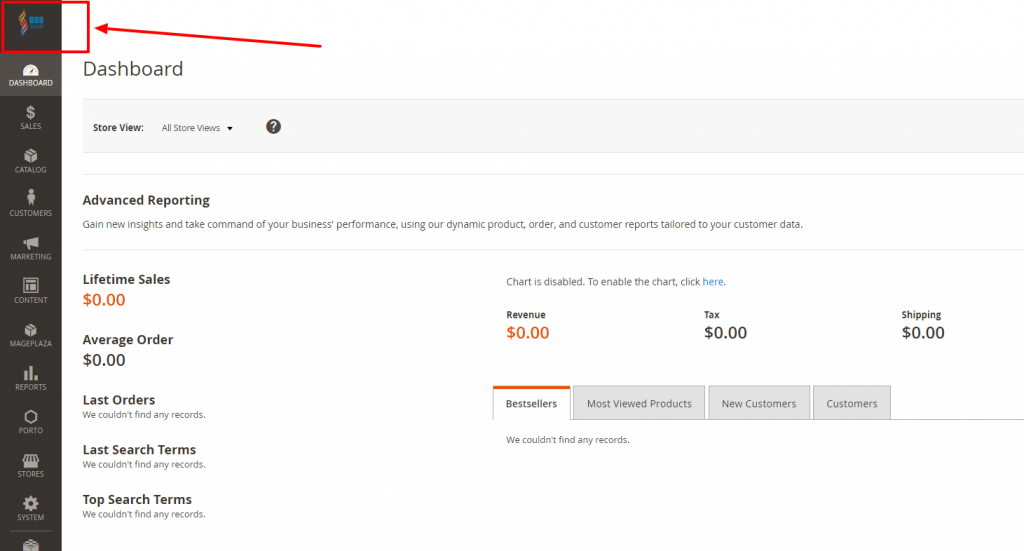**Detailed Caption:**

This image displays a screenshot of a sales dashboard used for tracking product sales. In the top left corner, there's an icon resembling a DNA swirl, labeled with "BSS" in blue text. Below "BSS," smaller text is visible but illegible, all enclosed in a red square with an arrow pointing to this icon within the left-side navigation directory. 

The navigation panel includes several options: Dashboard, Sales, Catalog, Customers, Marketing, Content, Mage Plaza, Reports, Porto, Stores, System, and one more cut-off description. "Dashboard" is the currently selected option.

The main screen is headed with the title "Dashboard" and features a gray banner below it reading, "Store View: All Stores" with a dropdown menu and a black circle containing a white question mark. Underneath, the heading "Advanced Reporting" is displayed in bold black text, accompanied by a gray description, "Gain new insights and take command of your business performances using our dynamic product, order, and customer reports tailored to your customer data."

Below this description, several key performance indicators are listed:

- Lifetime Sales: $0.00 (in orange)
- Average Order: $0.00
- Last Orders
- Last Search Terms
- Top Search Terms

Each of these metrics is followed by a note stating, "We couldn’t find any records."

To the right, there's a message stating, "Chart is disabled. To enable chart, click here," with "click here" as a blue hyperlink.

Further down, additional financial metrics are outlined:

- Revenue: $0.00 (in orange)
- Tax: $0.00 (in black)
- Shipping: $0.00 (in black)

Beneath these metrics, three tabs are present: Best Sellers, Most Viewed Products, and New Customers with "Best Sellers" selected. Below this tab in gray text, it states, "We couldn't find any records."